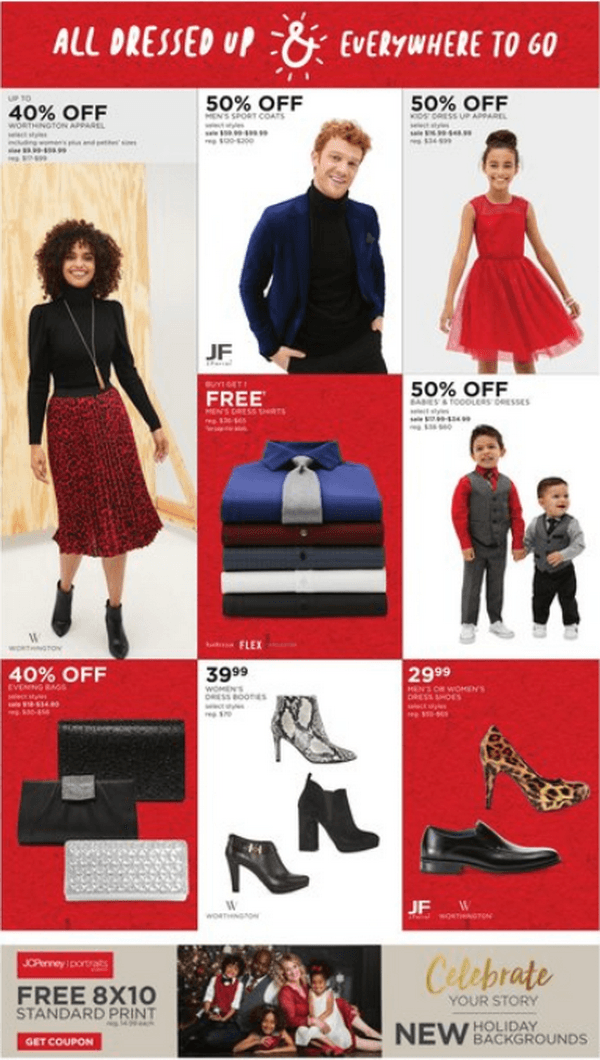### Captivating Deals for a Fashionable Holiday Season

The shopping website greets users with a vibrant red and white border at the top, where the catchy slogan "All dressed up & everywhere to go" is prominently displayed.

#### Featured Offers:
1. **Women's Apparel:** On the left side, a stylish woman is showcased wearing a long-sleeved black shirt, a red skirt, and black boots, with a banner above her highlighting "40% off".

2. **Men's Clothing:** Next to her, a man is seen in a sleek blue jacket over a black turtleneck, available at "50% off".

3. **Women's Dress:** To the right, a young woman with a bun is elegantly dressed in a sleeveless red dress, also marked "50% off".

4. **Men's Dress Shirts:** Centrally positioned is a neatly stacked collection of men's dress shirts.

5. **Children's Suits:** Further right, two young boys appear dapper in their suits, offered at "50% off".

#### Accessories & Footwear:
1. **Bags and Wallets:** The bottom row kicks off with a stylish bag paired with three wallets (two black, one silver), all tagged "40% off".

2. **Boots:** Adjacent to this display are three pairs of boots priced at $39.99—two in black and one in a striking black and white pattern.

3. **Footwear Specials:** To the right, contained within a red square, is an enticing deal featuring an animal print stiletto and a pair of men's black shoes, both priced at $29.99.

#### Special Promotion:
1. **Free Print Offer:** In the bottom row, a graphic advertises a "free 8x10 standard print" with a coupon.

2. **Holiday Backgrounds:** Accompanied by the phrase "Celebrate your story, new holiday background," this section features a heartwarming picture of a family.

### Embrace the season with these fantastic offers and dress up for every occasion with style and savings!